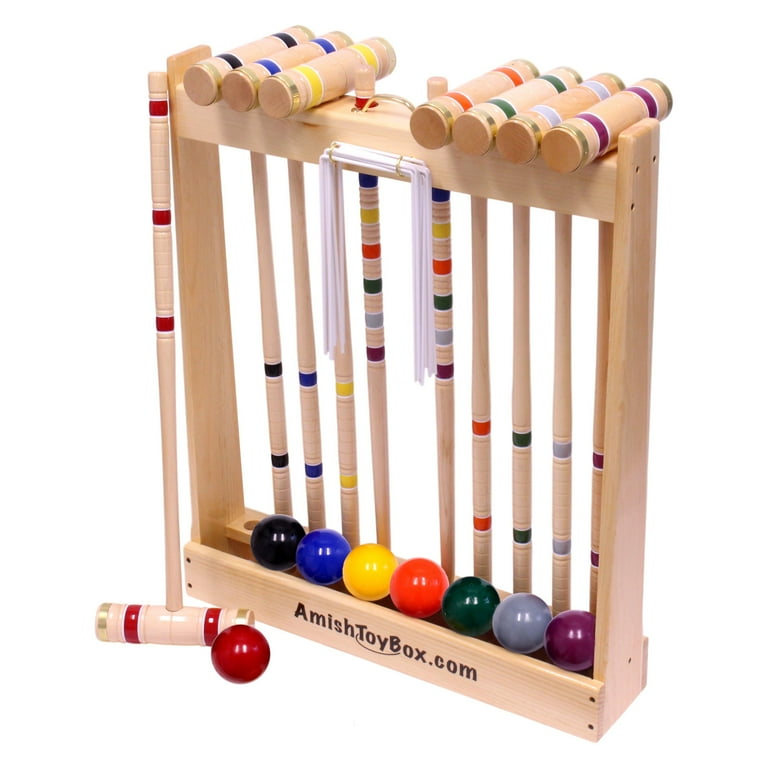This professionally taken, close-up photograph showcases a beautifully made croquet set against a pristine white background, making every detail stand out sharply. The set is framed by a light brown, polished pine wooden rack emblazoned at the bottom with the brand name, AmishToyBox.com. The rectangular rack supports eight mallets, each adorned with colorful stripes on both the heads and handles. The colors — black, blue, yellow, orange, green, gray, purple, and red — correspond perfectly with a matching set of eight brightly colored balls lined up along the bottom of the structure. One red mallet and its companion red ball are placed outside the rack, leaning against it, adding a touch of casual arrangement to the structured presentation. Additionally, the set includes white metal wickets hanging on hooks attached to the frame, ready to be used in play. The entire composition of the image suggests a well-crafted and easily storable set, perfect for an elegant game of croquet.